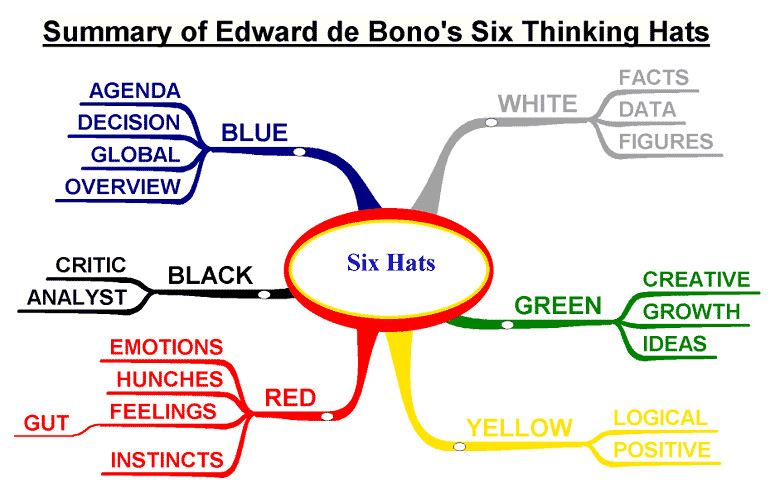The image is a simplistic, possibly MS Paint-created diagram that serves as a summary of Edward de Bono’s Six Thinking Hats. The diagram is centered around a red oval labeled "Six Hats," from which six color-coded branches extend, each representing a different mode of thinking in de Bono’s theory. Though roughly drawn and not very professional-looking, the visual gets the idea across effectively.

1. **Blue Branch:** Focused on agenda-setting and decision making, it includes sub-branches for Agenda, Decision, Global, and Overview.
   
2. **Black Branch:** Centers on critical thinking and analysis, branching into Critic and Analyst.
   
3. **Red Branch:** Associated with emotions and intuition, it lists Emotions, Hunches, Feelings, Gut Instinct, and Instincts.
   
4. **Yellow Branch:** Highlights optimistic and logical thinking, simply labeled Logical and Positive.
   
5. **Green Branch:** Represents creativity and growth, featuring Creative, Growth, and Ideas.
   
6. **White Branch:** Dedicated to facts and information, it includes Facts, Data, and Figures.

This interconnected web-like structure captures the multifaceted approach of de Bono’s Six Thinking Hats, offering a visual overview of the different cognitive styles—analytical, emotional, factual, and creative.